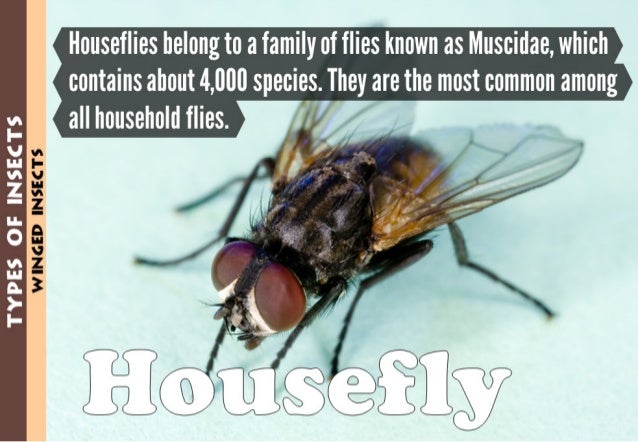This detailed image features a close-up of a housefly, clearly labeled "housefly" in white text at the bottom left with a thin black outline. The housefly is oriented looking down to the left, with clear wings, a gold-colored back, and maroon eyes. The background behind the fly is white. At the top of the image, a gray text box contains a description in white font stating: "Houseflies belong to a family of flies known as Muscidae, which contains about 4,000 species. They are the most common among all household flies." On the left side of the image, there are two vertical labels with text rotated 90 degrees: one is a brown bar with "types of insects" in white uppercase font, and the other is a peach or cream-colored bar with "winged insects" in black uppercase font. The overall background of the image is light turquoise. This image appears to be a section from a biology or science book, or possibly a detailed educational social media post.